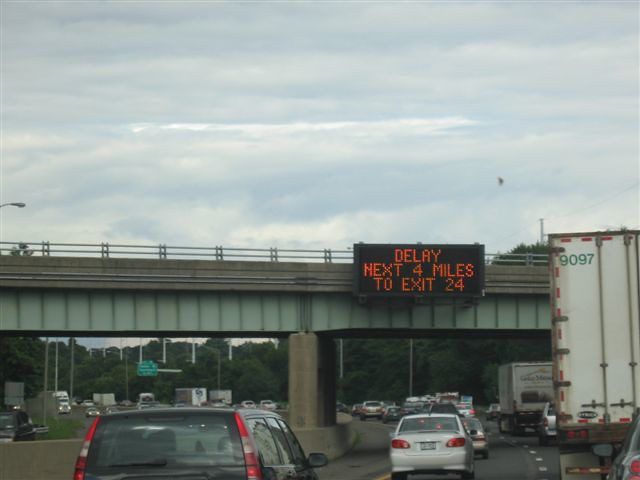This outdoor daytime photograph captures a busy, multi-lane freeway teeming with traffic, including cars, SUVs, and large semi-trucks. Prominently featured in the background is an overpass with a light-green metal sheet on its side, supporting a digital display that reads "Delay next 4 miles to exit 24." A distinct detail is the number "9097" visible on the back of one of the semi-trucks. The overpass, equipped with a railing and an inactive streetlight, looms above the three clearly discernible lanes of highway traffic, suggesting a hectic and congested scene. Surrounding the highway are tall trees, and the sky is blanketed with clouds, adding a somber tone to the image. The vantage point appears to be from someone leaning out of a car window, providing a first-person perspective of the traffic ahead, which includes various vehicles in different lanes.